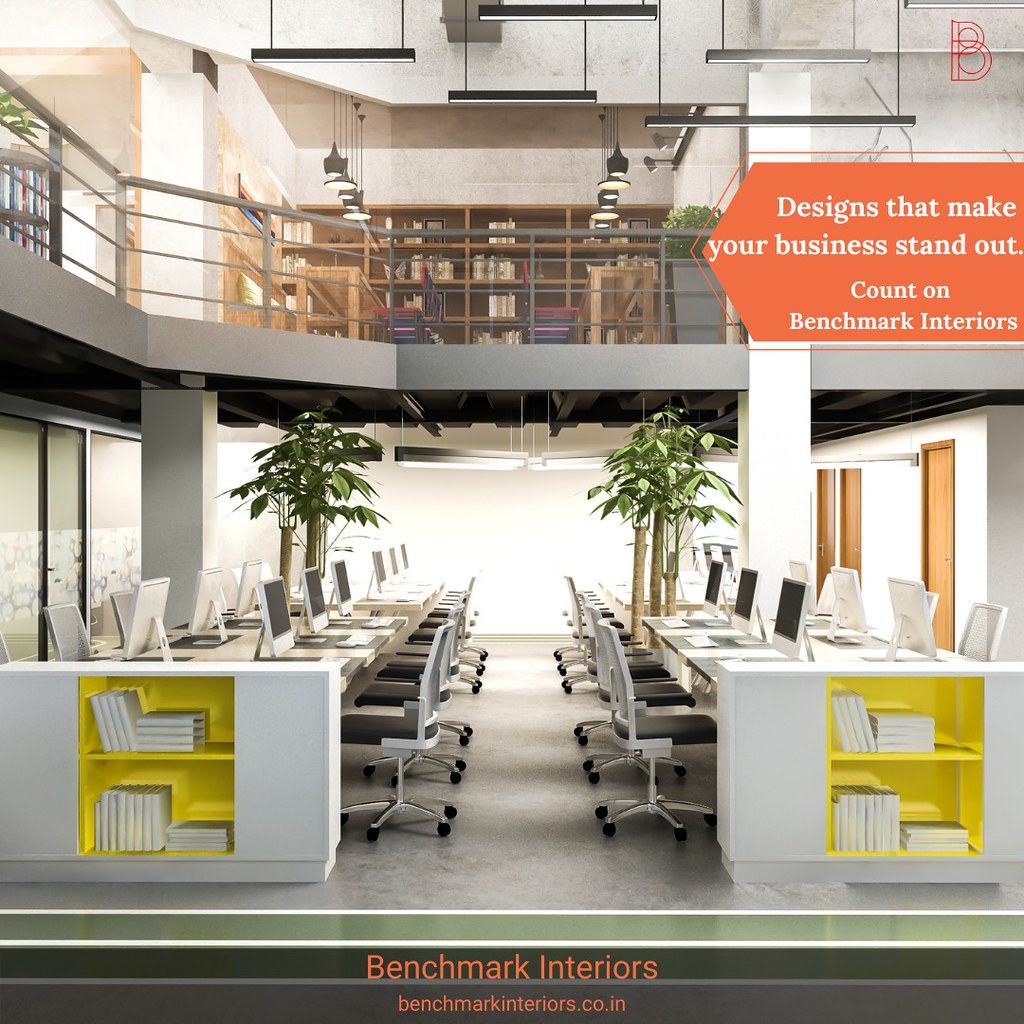This advertisement for Benchmark Interiors, a company specializing in interior design, features a meticulously crafted workspace displayed in a realistic, computer-generated image. The setting is an open, two-story office with a modern, industrial aesthetic. On the top floor, accessible behind a gray metal railing, are multiple seating areas equipped with wooden tables and bookshelves filled with books, all illuminated by drop-down fluorescent lights set in black fixtures.

The bottom floor showcases a professional environment with two long rows of Apple iMac computers complete with wireless keyboards and magic mice. Each workstation includes a swivel chair, set up for efficiency and comfort. Additionally, there are numerous cabinets holding manuals and loose-leaf binders in yellow cubby holes. The dark ceiling overhead accentuates the industrial look with its hanging warehouse-style lamps. A revolving cabinet on the left also stores more binders, adding a touch of dynamic functionality.

The advertisement text, prominently placed, states: "Designs that make your business stand out. Count on Benchmark Interiors." The company's logo and website, benchmarkinteriors.co.in, are highlighted in orange text at the center bottom of the image. Overall, the advertisement effectively emphasizes the modern, attractive, and highly functional workspace designed by Benchmark Interiors.